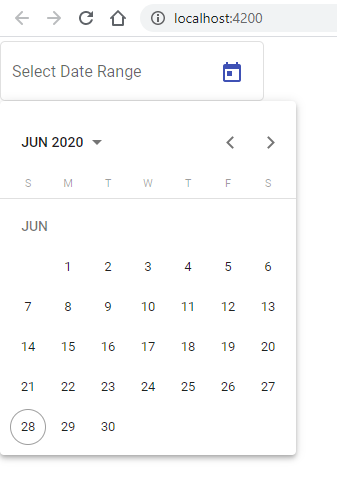Screenshot of a Phone Displaying a Calendar Application

The screenshot, taken in portrait orientation, reveals a calendar application on a smartphone. The image lacks defined external borders and exhibits a thin grey bar running horizontally at the very top, separating the search bar from the rest of the page. The top bar hosts two inactive-looking grey arrows pointing left and right, presumably for navigation, followed by a refresh icon and a home icon. Below this top bar is a grey-like information strip featuring a circle with an eye icon and the text “localhost:4200” in black and grey font, respectively.

Just beneath this information strip, a narrow grey box contains the text “Select date range” in grey, accompanied by a blue calendar icon on the right. This setup rests against a white background.

The central focus of the image is a calendar displayed with a slight shadow effect, giving it a subtle 3D appearance. The calendar header indicates the month as "June 2020," located in the top left corner. Adjacent to this label is a drop-down caret, and to the right of it are navigation arrows allowing the user to toggle between months. The calendar grid starts on Monday, June 1st, and ends on Tuesday, June 30th. Notably, Sunday, June 28th, is circled in grey, signifying a possible event or note on that date.